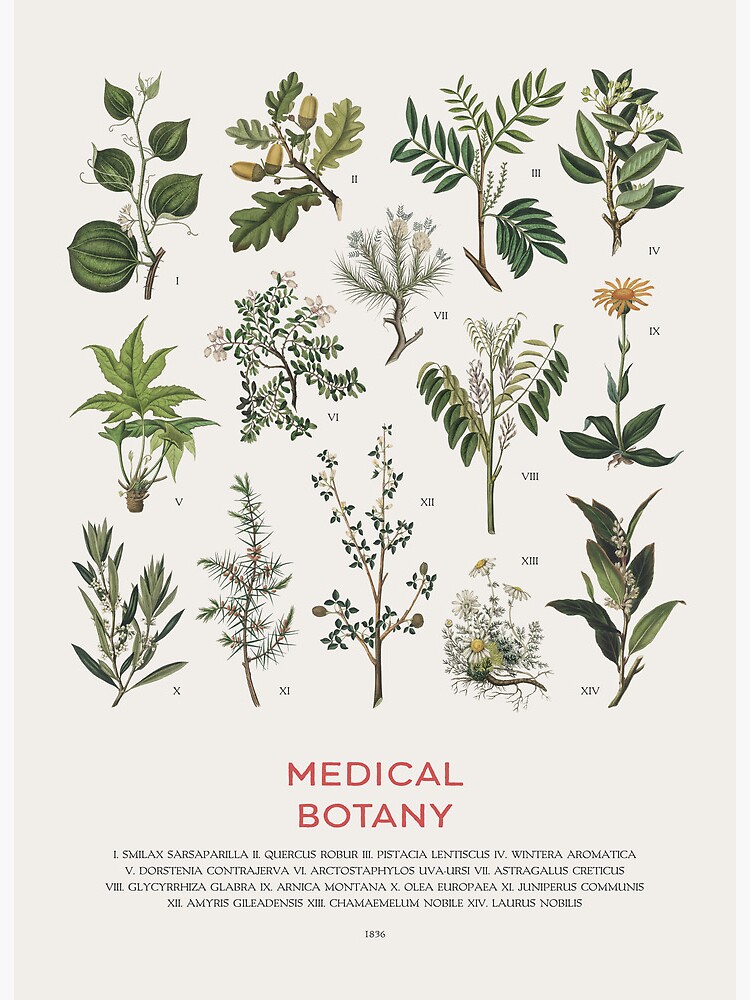The image is a detailed, colored drawing illustrating various plants central to medical botany. It features a white background with meticulously drawn and colored plants, each labeled with Roman numerals I to XIV. Each plant depiction includes branches, leaves, flowers, acorns, and sometimes pods or stalks, colored naturally—green leaves, beige acorns, and multicolored flowers and pods. In the center bottom of the image, the title "Medical Botany" is prominently displayed in red, with the year 1836 noted below. The plants include Smilax sarsaparilla, Quercus rober, Pistachia lenticus, Wintera ameratica, Dorstenia contravera, Arctostaphylos uva-ursi, Astragalus cretaceus, Glycyrrhiza glabra, Arnica montana, Olea europaea, Juniperus communis, Amaryllis belladonna (misidentified as Amaryllis gildianus in the original notes), Chamomilla nobilis (commonly known as Roman chamomile), and Laurus nobilis.